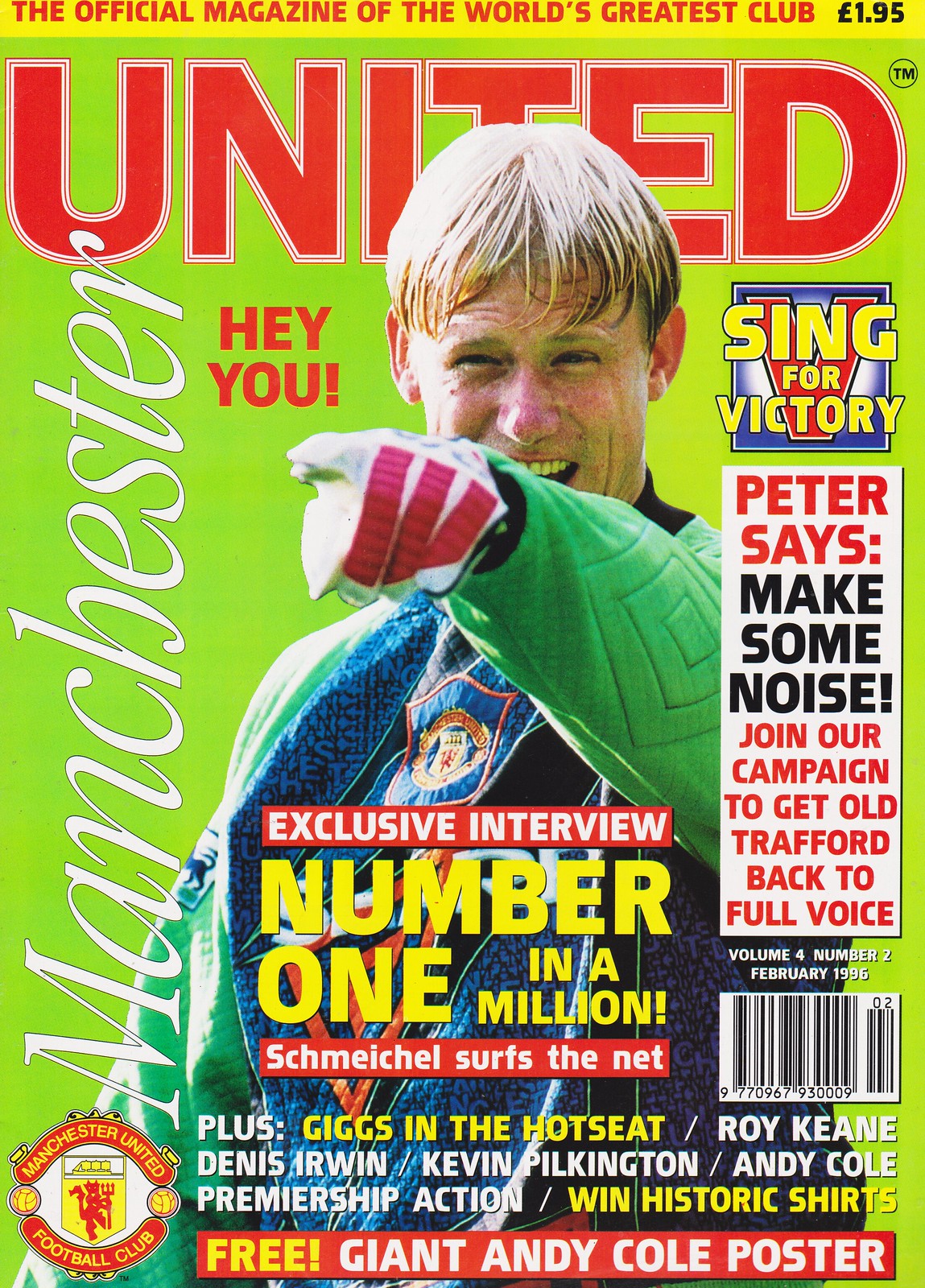The image depicts the cover of a sports magazine featuring a vibrant photograph of a football player positioned centrally against a yellow background. The player, who seems to be a goalkeeper identifiable by his gloves and sweaty hair clinging to his forehead, is animatedly smiling and pointing slightly leftward. His mouth is open as if he is shouting or celebrating. The top of the cover reads, "The official magazine of the world's greatest club," rendered in white text, emphasizing the magazine's association with Manchester United. Just below, the title "United" stands out in bold red text with a contrasting white border. Additional details include phrases like "Exclusive interview number one in a million," "Schmeichel serves the net," and "Sing for victory, Peter says, make some noise, join our campaign to get Old Trafford back to full voice." The cover employs a diverse color palette with shades of yellow, red, green, black, white, blue, and orange, adding to its dynamic appeal.